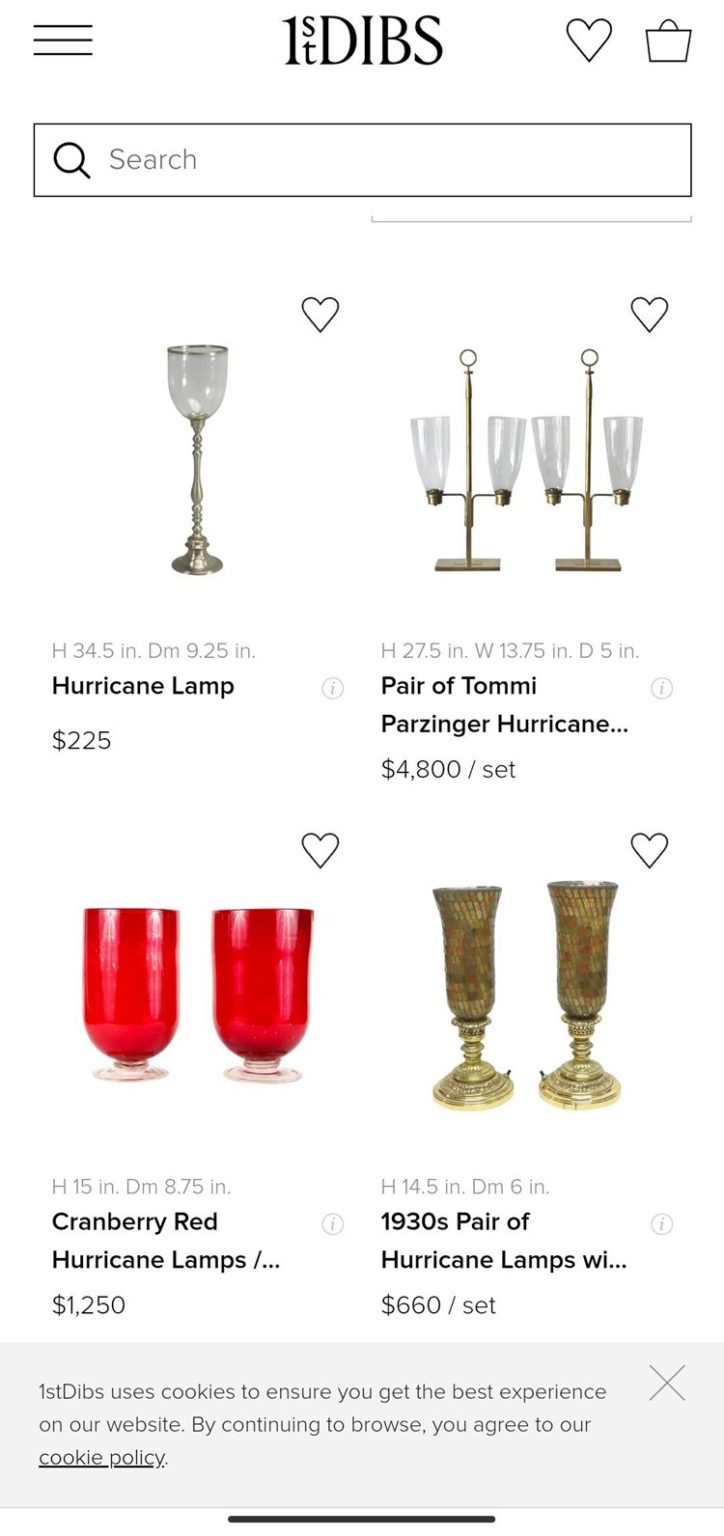This screenshot showcases an e-commerce mobile application with a clean, white background. On the top left corner, there is a 'hamburger' menu icon that can be clicked for additional information. In the center, a charming logo spells out "First Dibs," creatively incorporating a number "1" next to an "S" placed over a "T," followed by the capital letters "D-I-B-S." To the right of this logo, there is a heart icon for liking items, and a shopping basket or cart for purchasing. Below these icons, a search bar enables users to find specific products.

Users can interact with the displayed products by clicking on the hearts in front of each listing to "like" them. Detailed listings are present, including:

1. A single hurricane lamp priced at $225.
2. A luxurious pair of Tommy Parzinger hurricane lamps, available for $4,800 per set.
3. Cranberry Red hurricane lamps, standing 15 inches high with a diameter of approximately 8.75 inches, priced at $1,250.
4. A unique 1930s pair of hurricane lamps in a greenish-gold color, priced at $660 for the set.

The overall impression is that of a high-end website offering a range of exquisite and expensive lighting options.